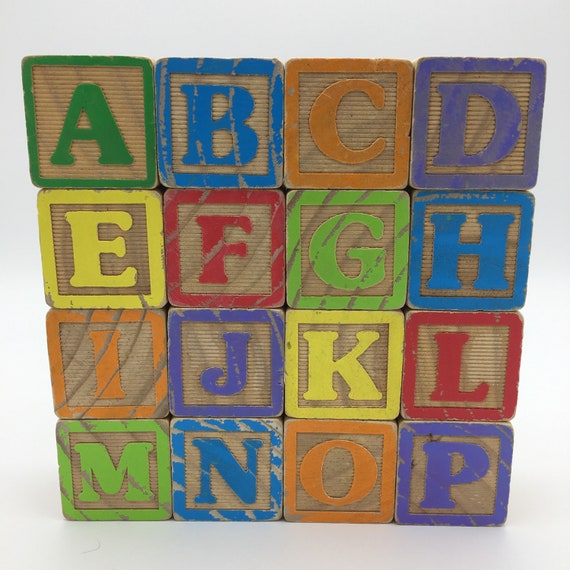This close-up photograph captures a set of vintage wooden alphabet blocks, arranged in a neat 4x4 grid against a plain white background. Each block features a carved letter of the alphabet, painted in vibrant colors with a matching colored border. From top to bottom, left to right, the blocks display the letters A to P: the first row includes a green A, blue B, orange C, and purple D; the second row shows a yellow E, red F, green G, and blue H; the third row contains an orange I, purple J, yellow K, and red L; and the last row features a green M, blue N, orange O, and purple P. The blocks exhibit signs of wear, with scuffed paint and rugged edges, indicating they have been well-used and loved. The carved letters and borders are the colored parts, while the rest of each block remains wooden.